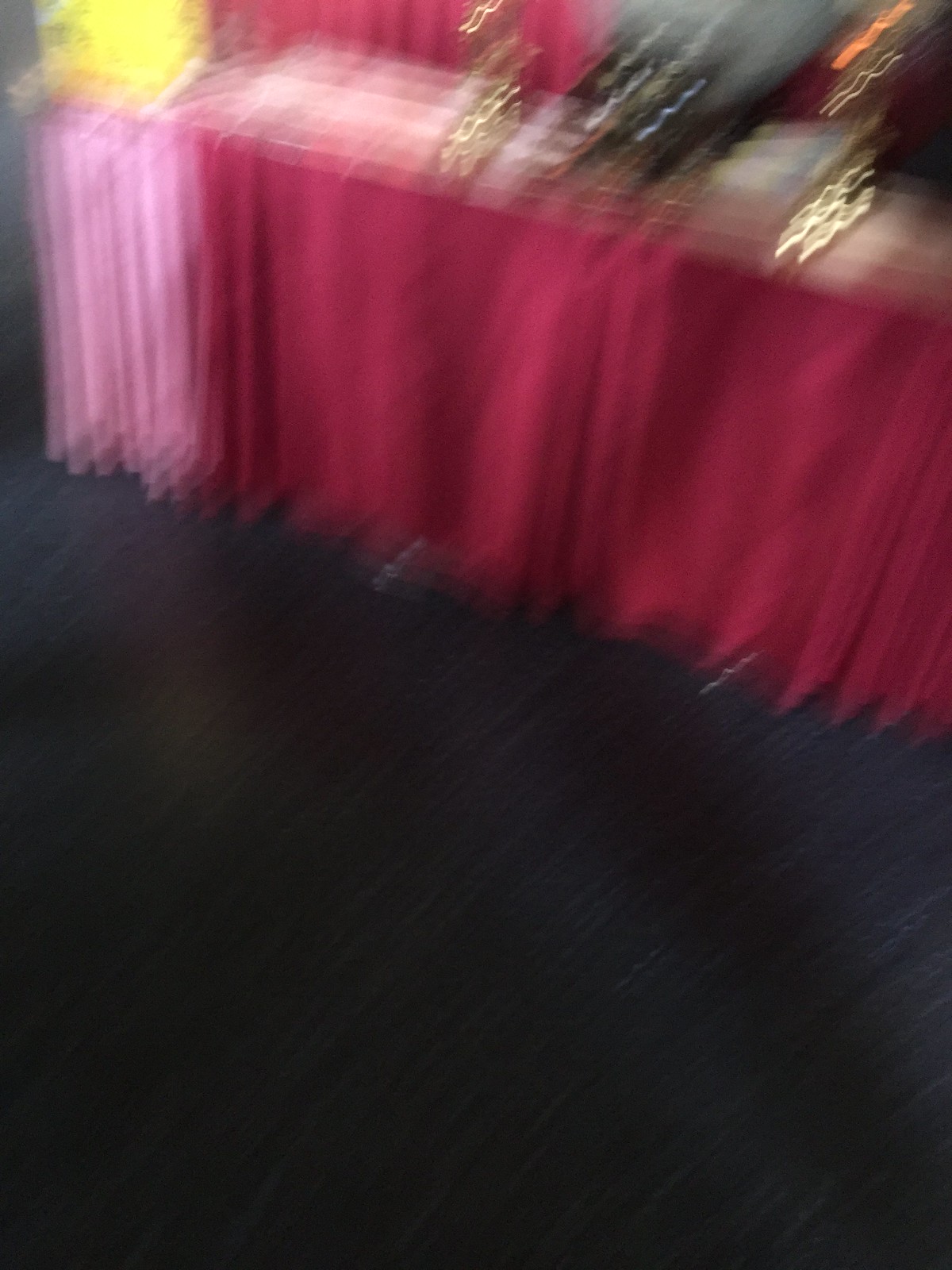The image is an extremely blurry photograph of what appears to be a retail area, likely a clothing store. Despite the lack of focus, one can identify racks filled with garments. Near the center and left side of the image, there are several items hung up in various shades of pink, resembling draperies but clearly suspended on hangers. To the right, a large collection of scarlet red items are also displayed on a rack. The presence of hangers and a sign positioned atop one of the racks further indicates the setting is a store. At the bottom of the image, there are indistinct dark shapes, possibly the feet of shoppers or more racks. Although the blurred quality obscures precise details, the overall scene hints at a busy retail environment showcasing a variety of clothing items on display.